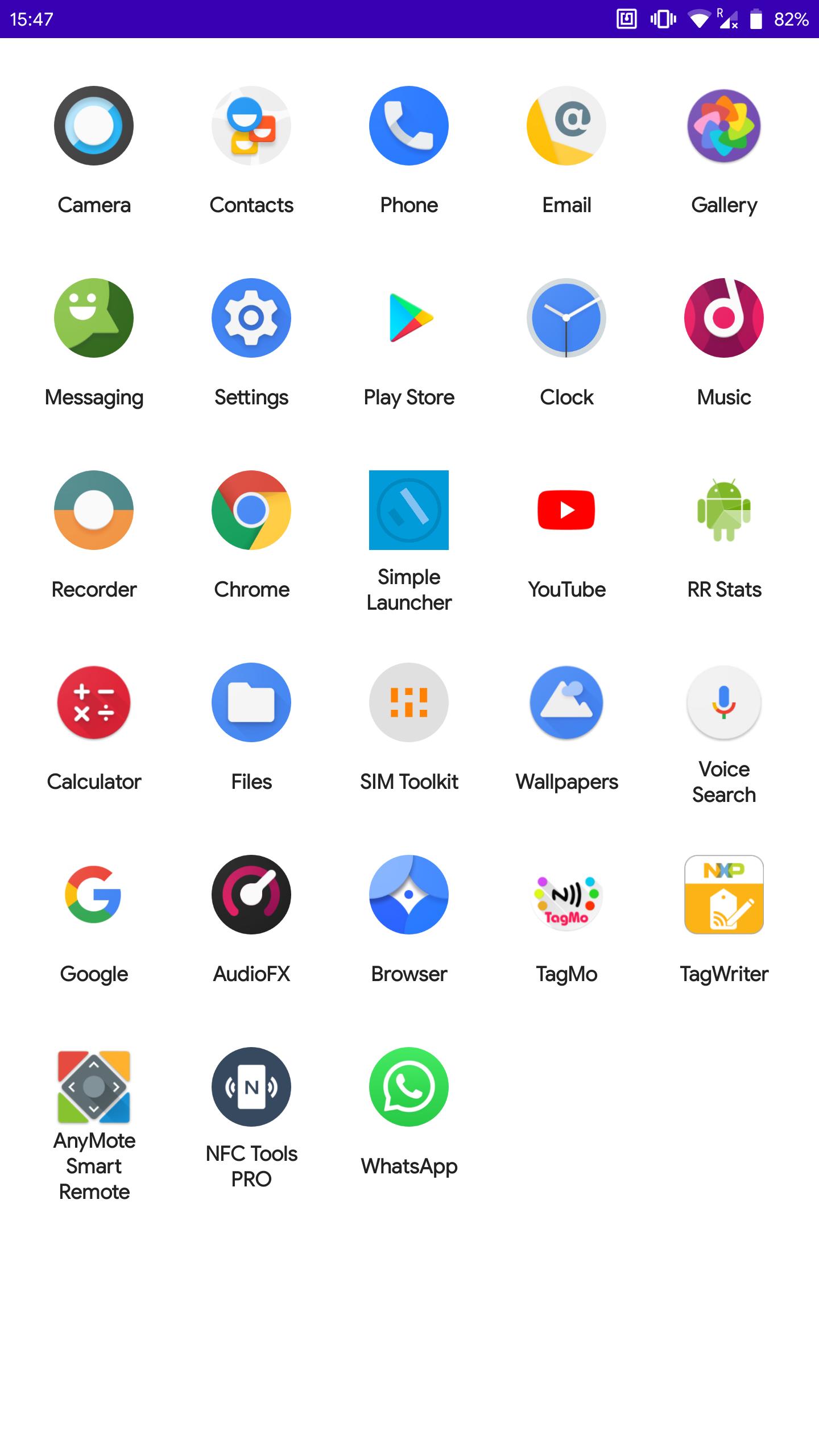The image depicts a smartphone home screen with a detailed layout of apps and icons. At the very top, a purple status bar displays the time as 15:47 on the left and the battery status, 82%, along with a vertical white battery icon on the right. 

Below the status bar is the first row of app icons which includes Camera, Contacts, Phone, Email, and Gallery. The Phone app is highlighted with a blue circle containing a white telephone icon. 

The second row features Messaging, Settings, Play Store, Clock, and Music. The Messaging app icon is distinguished by a green circle with a smiley face inside. 

The third row consists of Recorder, Chrome, Simple Launcher, YouTube, and RR Stats. The Calculator app is shown with a red circle above it while this row also includes Files, SIM Toolkit, Wallpapers, and Voice Search. 

On the fourth row, the iconic Google app is displayed with its logo 'G' colored in red, yellow, green, and blue. This is followed by Audio FX, Browser adorned with a blue circle, Tag MO, and Tag Writer.

The final row starts with Anymote Smart Remote, which is represented by a multicolored box above it, followed by NFC Tools Pro. Lastly, the row includes a green circle with a telephone icon, labeled as WhatsApp.